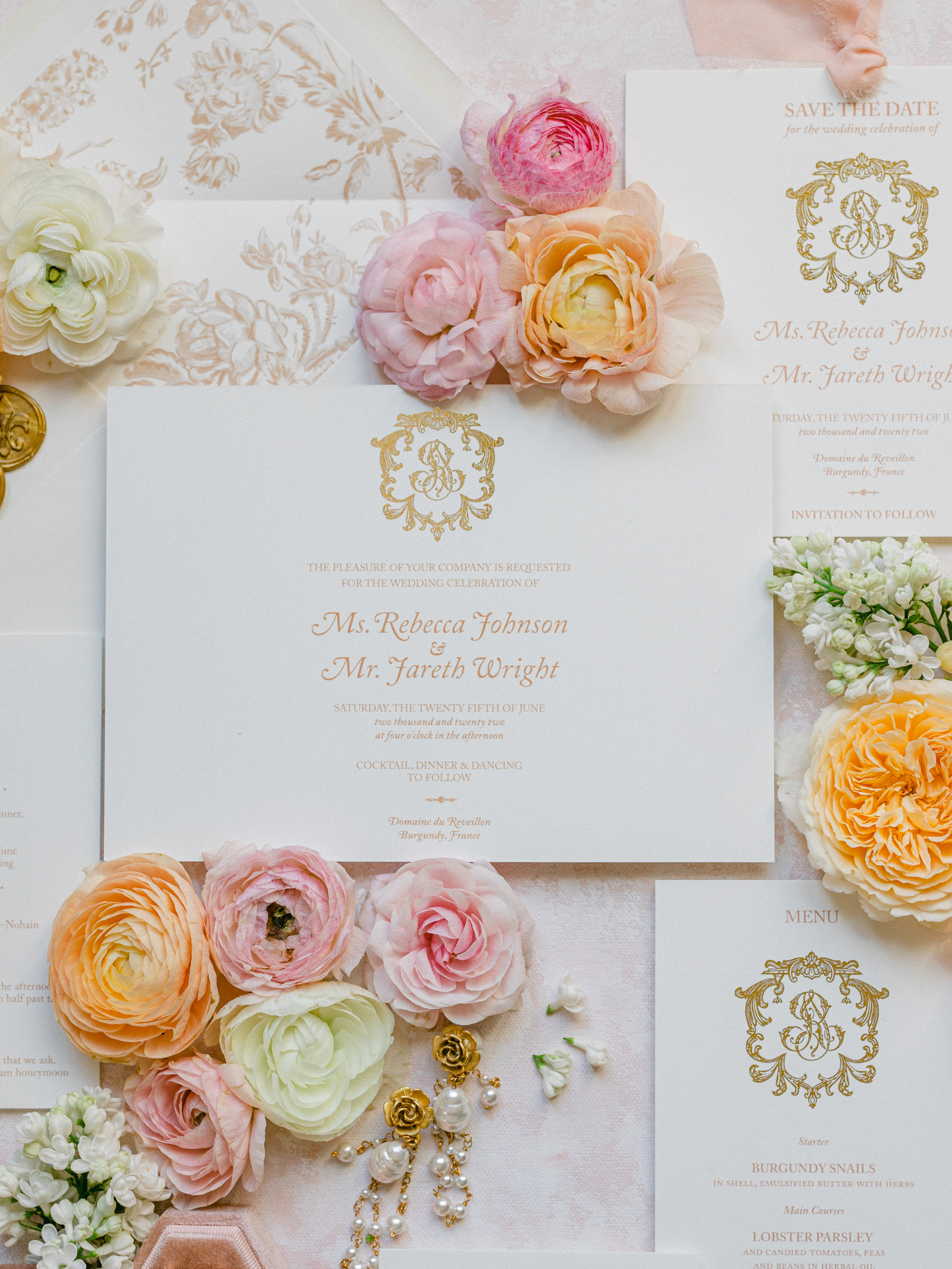This photograph features a detailed aerial view of a wedding invitation set elegantly arranged on a pastel-themed floral background. At the center lies a white rectangular wedding invitation card with gold-embossed text announcing the union of Ms. Rebecca Johnson and Mr. Ferrith White. Surrounding the invitation is a beautiful assortment of flowers, including light pink, orange, white, and purple blooms, some arranged as small individual blossoms and others more abundantly placed at the bottom. The scene is further accentuated by scattered pearls and delicate petals, adding a touch of sophistication. Accompanying the central invitation are additional cards featuring a "Save the Date" notice and a menu selection. A pair of gold earrings and a white baby beret are subtly positioned within the arrangement, contributing to the overall romantic and carefully curated aesthetic of the display.